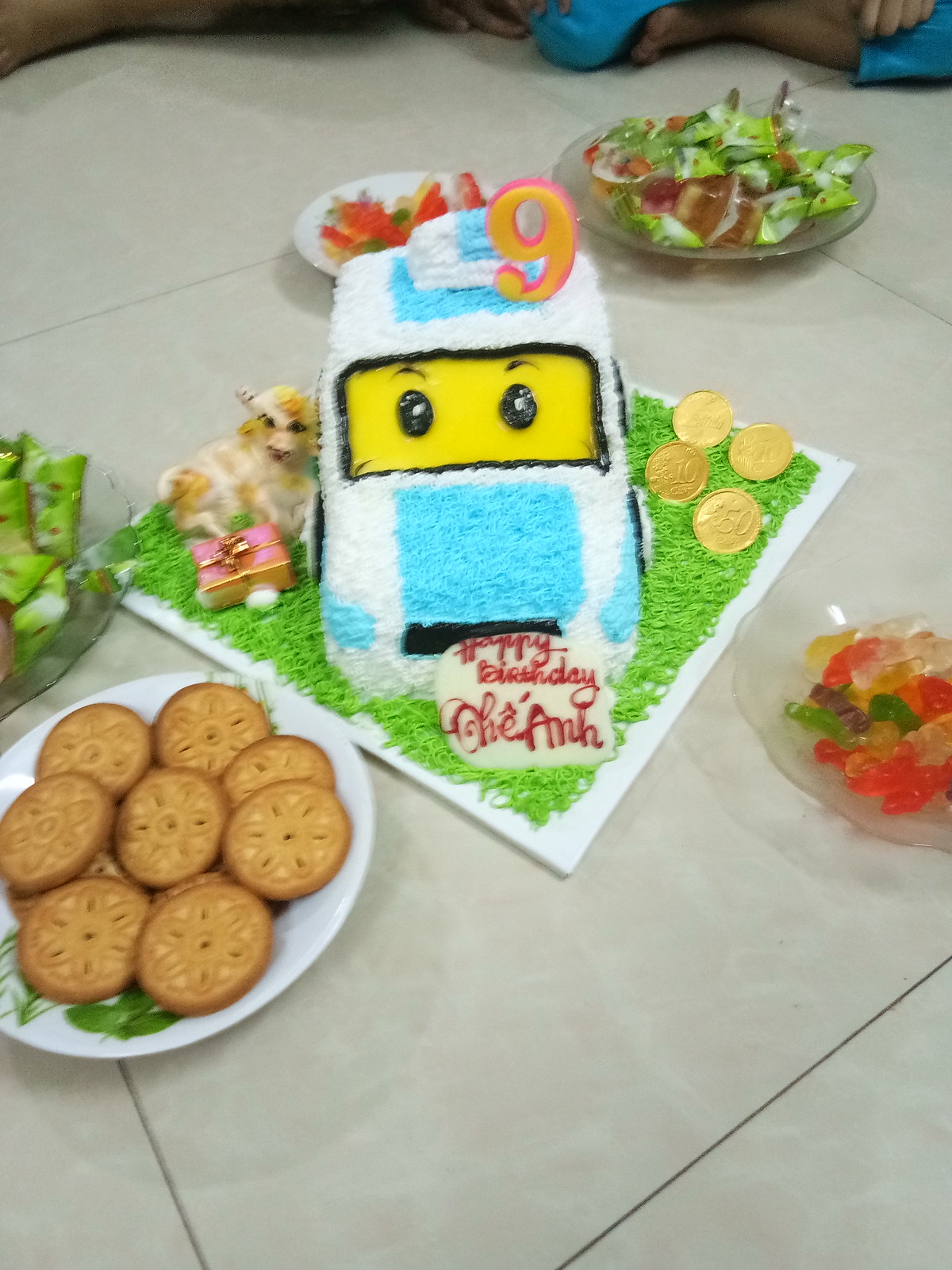The photograph captures an indoor setup for a child’s birthday celebration, centered around an intricate birthday cake designed to resemble a race car in white and blue icing. The cake features a yellow windshield adorned with black eyes and eyebrows, and a prominent number nine candle on top. The inscription on the cake reads "Happy Birthday Che On," and green icing is creatively piped around the cake to simulate grass. The cake rests on a square white surface, surrounded by various festive elements. 

To the right of the cake, there is a glass dish containing wrapped candies. On the left, a small pink gift and a toy animal are placed near four gold foil chocolate coins. Additionally, a white plate holds brown cookies with floral designs, and there are glass trays with gummy bears and gummy worms. In the background, slightly cut off at the edges, you can see the feet and hands of a child, adding a subtle yet personal touch to the celebratory scene. The entire arrangement is set atop large, beige ceramic tile flooring.